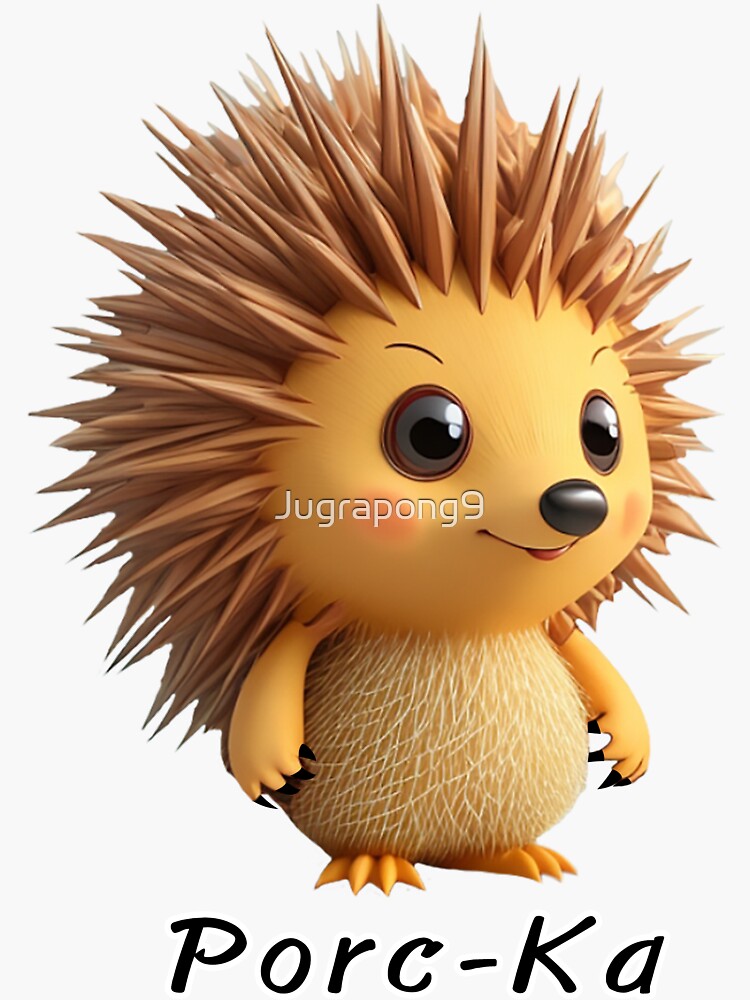The image showcases a 3D-rendered, computer-generated porcupine named "Porca," set against a solid white background. Porca is depicted with a chubby, short, and stubby body, featuring a gold-colored, slightly yellowish skin tone. His cute, cartoon-like face is adorned with glossy black eyes, a black nose, slight pink cheeks, and a cheerful smile with a little tongue sticking out. Quills radiate from Porca's head and back, clearly indicating his porcupine nature, while his belly exhibits a lighter brown, fuzzy texture. His arms and feet, which are also yellowish, have several tiny toes. Porca stands facing to the right at a slight twisted angle. Below the character, the name "Porca" is written in a foreign language as "P-O-R-C-K-A," and there is a watermark that reads "Jugrepong 9."